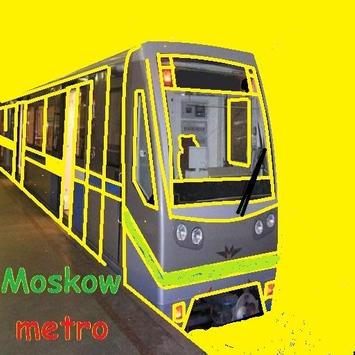This image is a digitally edited illustration of a Moscow Metro train car and platform. The central focus is the front of the train car, positioned slightly to the left. The train car itself features a vibrant mix of gray, lime green, yellow, blue, and red colors, with yellow lines outlining the windows, doors, and other sections. The background is predominantly yellow, adding a lively contrast. The text "MOSCOW METRO" is prominently displayed in the bottom left corner, with "MOSCOW" in green and "METRO" in red. Below the text, there is a platform shaded in gray and brown tones. The style of the image resembles a digitally modified illustration, with some elements appearing as though edited in Microsoft Paint, giving it a distinctive poster-like quality.